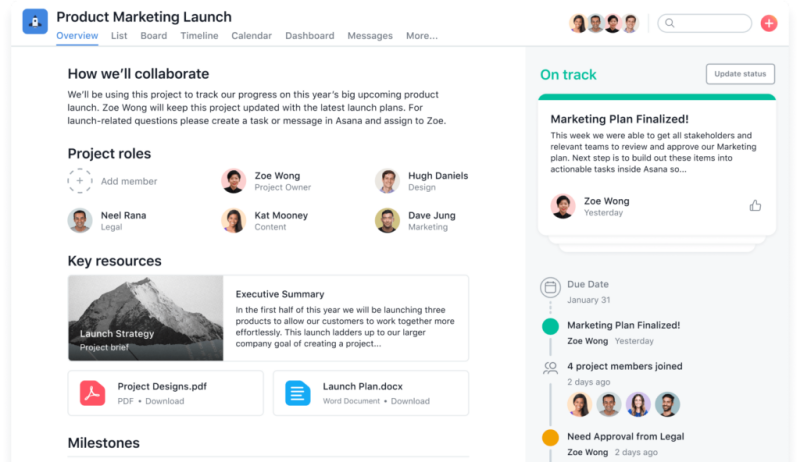A meticulously organized product marketing launch overview is displayed, highlighting several key project management tools and their respective functions. The interface, set against a predominantly white background, features various sections such as the list, board, timeline, calendar, dashboard, and messages, all accentuated in blue for clear visibility. The top of the image showcases four profile icons, presumably representing team members, two females and two males, who appear to be of Caucasian descent.

Adjacent to these profiles is a search bar with a magnifying glass icon and a plus symbol encased in a small red circle. An instructional segment titled "How We'll Collaborate" outlines the project’s goals and collaboration methods, emphasizing that Zoe Wong will keep the project updated with the latest launch plans. For launch-related queries, team members are instructed to create a task or send a message via Asana and assign it to Zoe.

A notable green-highlighted status update reads "On Track," with a marketing plan finalized by Zoe Wong. She mentions that this week’s focus is to have all stakeholders and relevant teams review and approve the marketing plan. The next step involves converting these strategies into actionable tasks within Asana.

Details of the project roles are exhibited, listing team members Neil Reyna, Zoe Wong, Kat Mooney, Hugh Daniels, and David Chung, indicating a team composition of predominantly men with possibly two women. A plus symbol invites the addition of new members.

Key resources and milestones are delineated, accompanied by a crucial due date set for January 31st. Recent updates include Zoe Wong’s finalized marketing plan post from the previous day and the inclusion of four project members needing legal approval from Zoe, noted as having been posted two days ago.